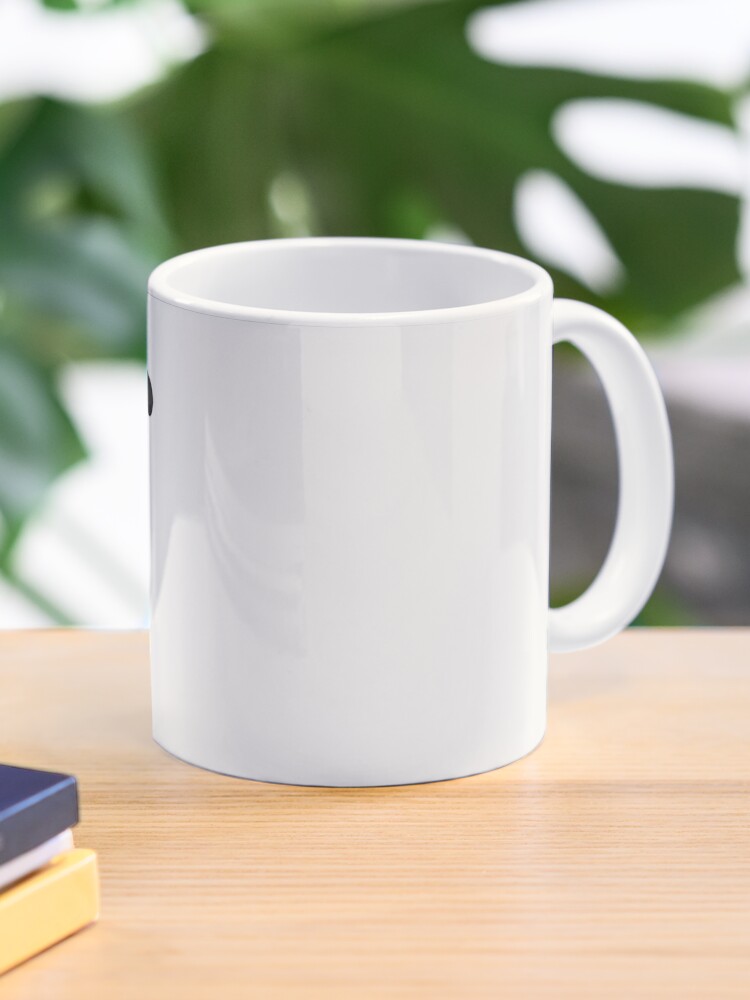This photograph captures a minimalist scene of a white ceramic coffee mug resting on a light brown wooden table. The mug, positioned with its handle pointing to the right, appears to have some sort of black mark or design on its left side, though the details are not clear. The table, seemingly brand new and clean, serves as the base for both the mug and a stack of books visible on the bottom left corner of the image. The books are layered in colors: the bottom one is yellow, the middle is white, and the top is dark blue. In the background, which is purposely blurred to highlight the mug, there are glimpses of greenery and patches of light, suggesting the presence of plants and possibly an outdoor setting. The overall simplicity of the composition, with its clean lines and soft lighting, gives the image a serene and contemplative atmosphere.